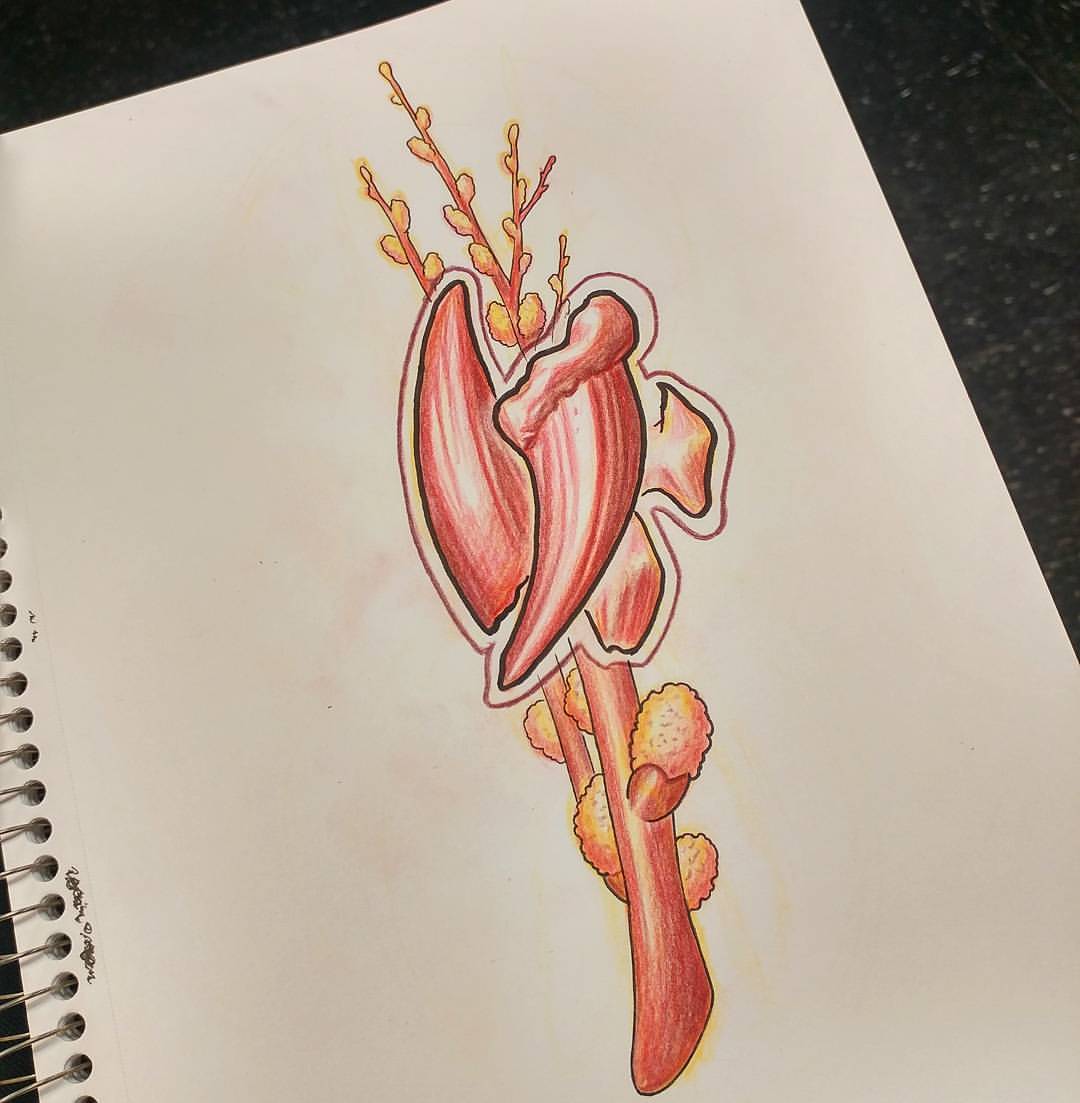The illustration is presented on a white notepad, bound along the left edge with multiple rings. The top-right corner of the notepad is distinctly black, providing a striking contrast. At the center of the notepad is a detailed drawing of an alien plant. The plant features a vibrant red stem that anchors the composition. Flanking the stem on both the left and right are clusters of yellow fluffballs. 

Prominently in the middle of the plant is a peculiar element resembling a broken canine tooth, adding an intriguing focal point to the illustration. To the left, the tooth appears to be flipped vertically, extending upwards and downwards. Branching out to the right are budding formations, indicative of the plant's growth.

Ascending towards the top of the illustration, the plant sports thin, delicate branches adorned with additional yellow floofs, giving the appearance of an otherworldly blossom. Interwoven in the design are shades of yellow and dark red, adding depth and complexity to the artwork.